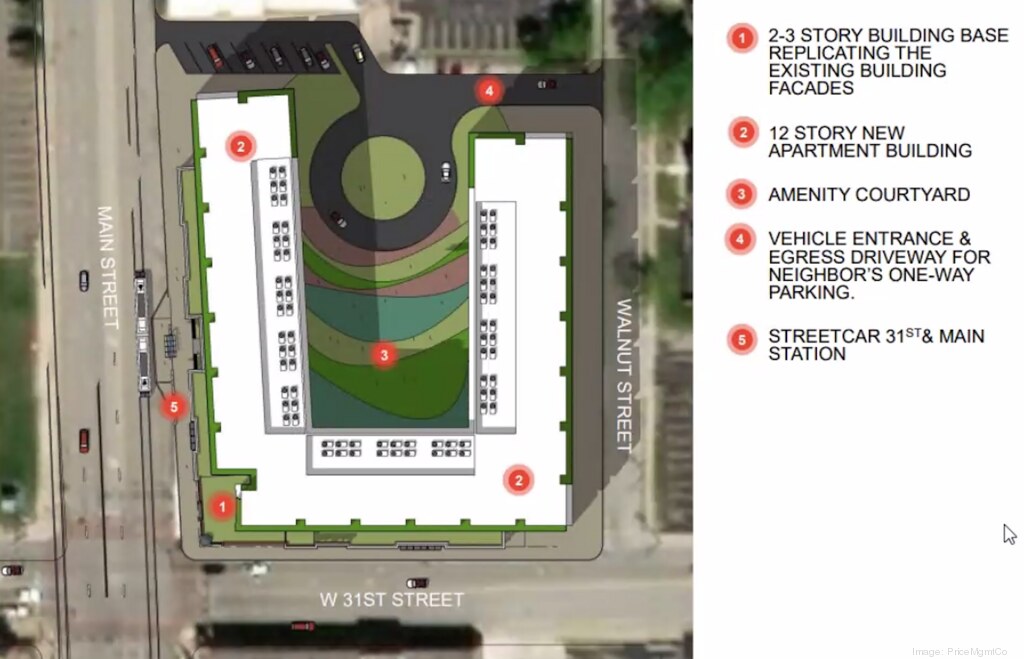This image depicts an overhead map featuring the layout of a new apartment complex situated between Main Street to the left, Walnut Street to the right, and West 31st Street at the bottom. The focal point is a building structure with an L-shaped design that includes several distinct areas, each marked by numbered red dots corresponding to a key located on the right side of the image. 

The legend defines these areas as follows: 
1. A two to three-story building base that replicates the existing building façades.
2. A new 12-story apartment building.
3. An amenity courtyard, centrally located within the layout.
4. A vehicle entrance and one-way egress driveway serving as parking access for neighboring properties.
5. A streetcar station at the intersection of 31st and Main Streets, facilitating public transit use.

Additionally, the map highlights a circular driveway at the entrance which directs vehicles to limited parking spaces, and it's complemented by abundant greenery, enhancing the visual appeal and potentially providing recreational space.